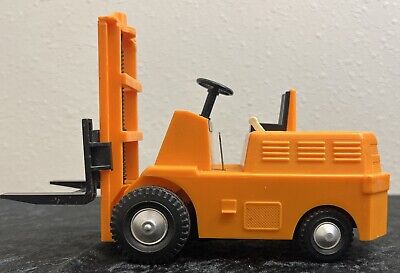The image features a tightly cropped, close-up shot of a plastic miniature forklift, designed either as a child's toy or a collectible item. The forklift is predominantly orange, accentuated with black components including the arms designed to lift heavy loads, the tires, the steering wheel, and the seat. It has two tires with silver hubcaps, where the front tire is larger than the rear one. The vehicle rests on what appears to be a black floor with white specks, contrasting against a white wall in the background. Additionally, there is a small white handle located next to the seat. The overall impression is that of a simplistic, non-professional photo focusing solely on the detailed toy forklift.